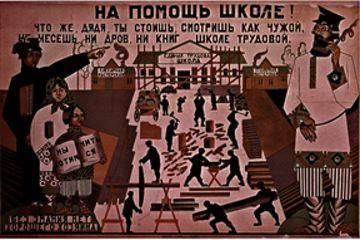This is a small, square image of a colorful vintage Russian poster with a sepia-toned palette that includes hues of pink, dark red, brown, cream, gray, black, and white. Featuring a brown background, the poster displays Russian text at the top, a headline in darker print, and additional Russian writing in the bottom left corner. 

The central portion of the image portrays a bustling construction scene with various laborers depicted as black silhouettes. These workers, engaged in manual tasks like carrying large beams, sawing wood, and hammering, populate a factory-like environment with building scaffolding and smoke-emitting chimneys in the background. 

On the left side, there is a commanding figure, likely an officer, pointing and appearing to give orders. Accompanying him are two women, one with a headscarf tied under her neck, and further below, two children in traditional dress; one child is holding two cans, while the other wears a flowery-bordered outfit.

On the right side of the poster stands a man with a thick black beard, dressed in a long white shirt and a black hat, speaking on a telephone with its coil stretching towards the top right corner.

Overall, this poster visually communicates a blend of authority and industriousness through its depiction of supervisory figures and diligent workers in a historical Russian revolutionary setting.